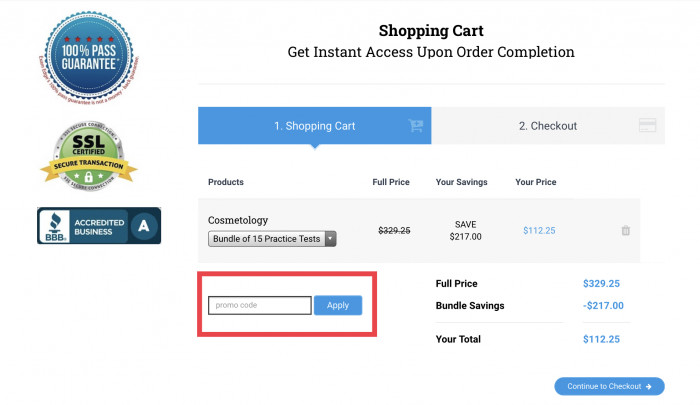The image is divided into two main sections. On the left-hand side, a vertical strip features three distinct circular badges. The top badge prominently displays "100% Pass Guarantee." Directly below it, the second badge signifies "SSL Certified Secure Transaction," indicating a secure and encrypted payment process. Completing the trio, the third badge features the Better Business Bureau logo, signifying an accredited business with an impressive A rating for reliability and trustworthiness.

To the right of this vertical strip, occupying the majority of the space, is the right-hand section titled "Shopping Cart." It emphasizes the immediate access provided upon the completion of an order. At the bottom left corner of this section, there is a text input box labeled for promo codes, accompanied by an "Apply" button to its right. Customers can enter a promotion code here to avail discounts, thereby reducing the displayed full price of $329.25.